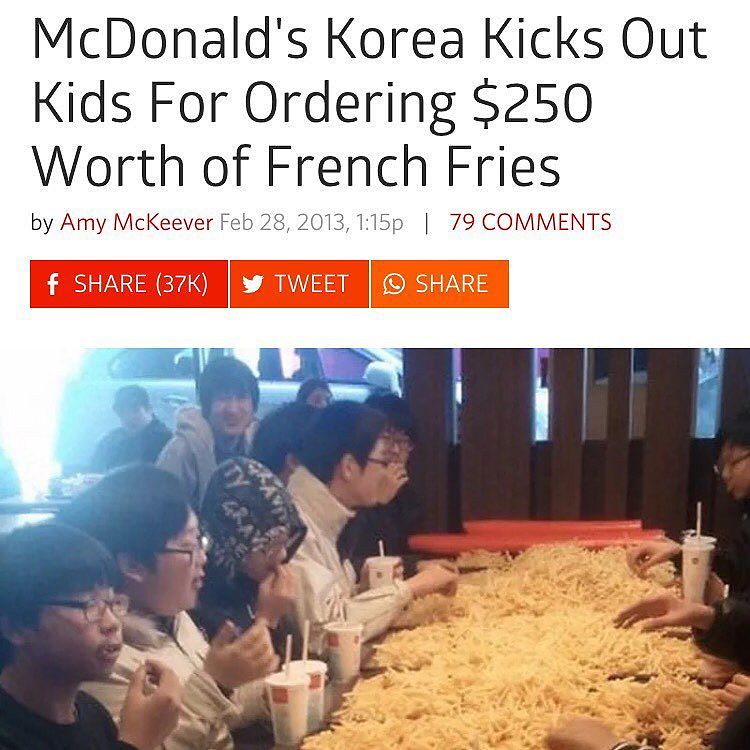The headline of the article is "McDonald's Korea Kicks Out Kids for Ordering $250 Worth of French Fries" by Amy McKeever, dated February 28, 2013, at 1:15 PM. The article, which has 79 comments, was widely shared with over 37,000 shares on Facebook and numerous tweets. The accompanying photograph shows a group of kids, primarily Asian, sitting inside a McDonald's restaurant at a table completely covered in French fries, piled about a foot high. There are at least five visible individuals, with some wearing black-rimmed glasses and a variety of clothing including a white jacket, black long-sleeved t-shirt, hooded sweatshirt with the letters "T-Y-N-G-R-A-V," a beige trench coat, and a black coat. The kids are actively eating the fries directly from the table, not using any plates, and have McDonald's cups in front of them. In the background, there is a visible group of additional people, wooden wall decorations, and windows through which a parked car can be seen.